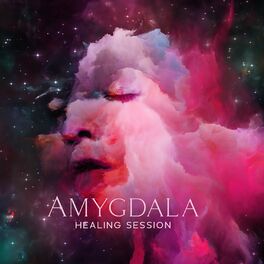The image presents an abstract representation of a person's face, primarily in pink hues tinged with white. The facial features, including closed eyes, a nose, and a dark mouth, are subtly blended into what appears to be a cloud-like material, with no distinct outline separating the face and neck from the background. The backdrop is a black, starry sky, speckled with white dots resembling distant stars. The overall scene invokes a deep space vibe, combining elements of outer space with ethereal, cloudlike formations. Below the face, text reads "AMYGDALA" in large letters, with "Healing Session" written underneath, suggesting the image might be an advertisement or poster, potentially for a meditative or therapeutic session.